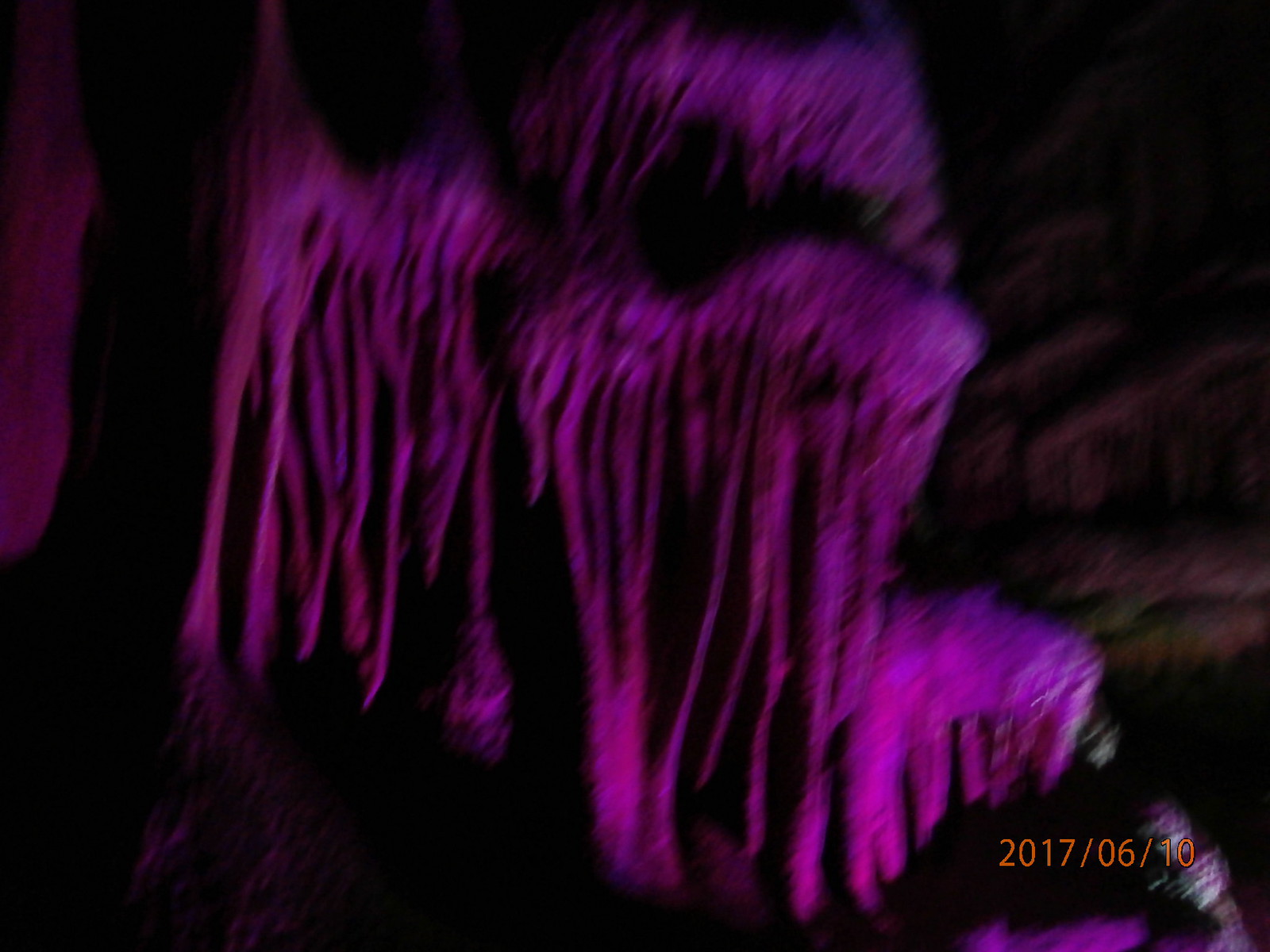Caption: 

"Captured on June 10, 2017, this intriguing photograph showcases a surreal scene resembling the mysterious innards of a cave. Dominating the left side of the image, a thick, purple substance appears to be melting and dripping down, creating a mesmerizing cascade. This purple mass extends from the top of the frame to just beyond the middle, lending a sense of depth and fluidity to the composition. Adjacent to this vivid purple, a stark black stripe runs vertically, possibly indicating a boundary or a shadow within the scene. In the background, earthy brown tones provide a contrasting backdrop, enhancing the enigmatic allure of the purple and black elements in the foreground. The overall effect is both strange and captivating, leaving much to the imagination about the true nature of this striking visual phenomenon."